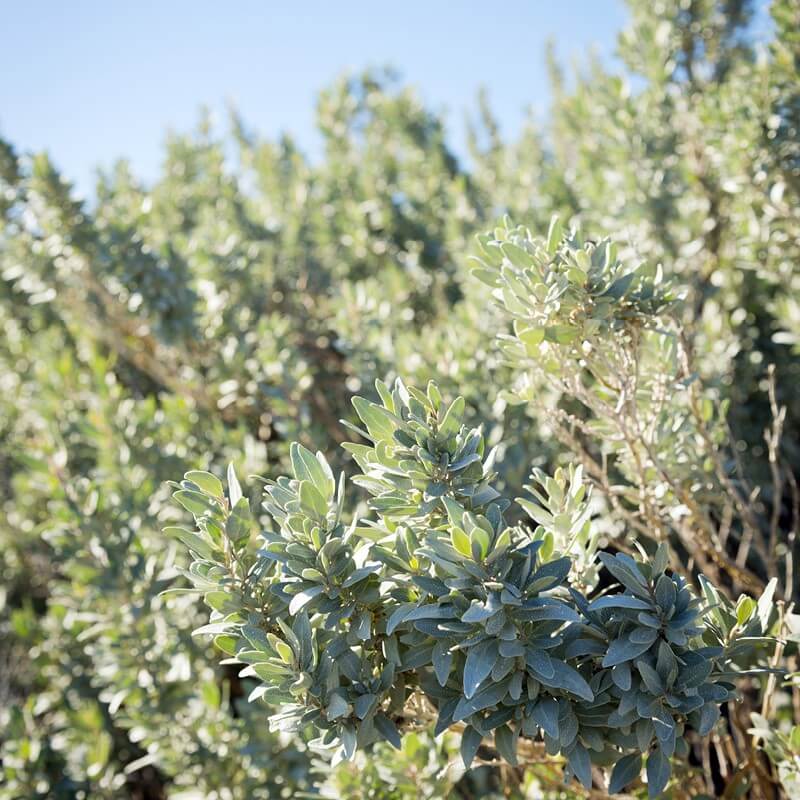This detailed photograph captures a close-up of lush, green leaves on a bush or tree in a square frame. The image showcases a striking contrast between the sharply focused central cluster of dark and light green leaves and the blurred background. In the lower right corner, you can discern some brown stems, which have tips touched with hints of light green or white. The central focus of the image is on this vivid cluster of leaves, surrounded by the soft blur of additional vegetation. Towards the top of the photograph, there’s a hint of blue sky and some indistinct, taller branches, which add depth to the scene. The left side of the image is also intentionally blurred, maintaining a seamless, natural gradient. The overall setting suggests a bright, sunny day, highlighting the vibrant greens against the blue sky backdrop. This composition emphasizes the rich textures and colors of the natural environment.